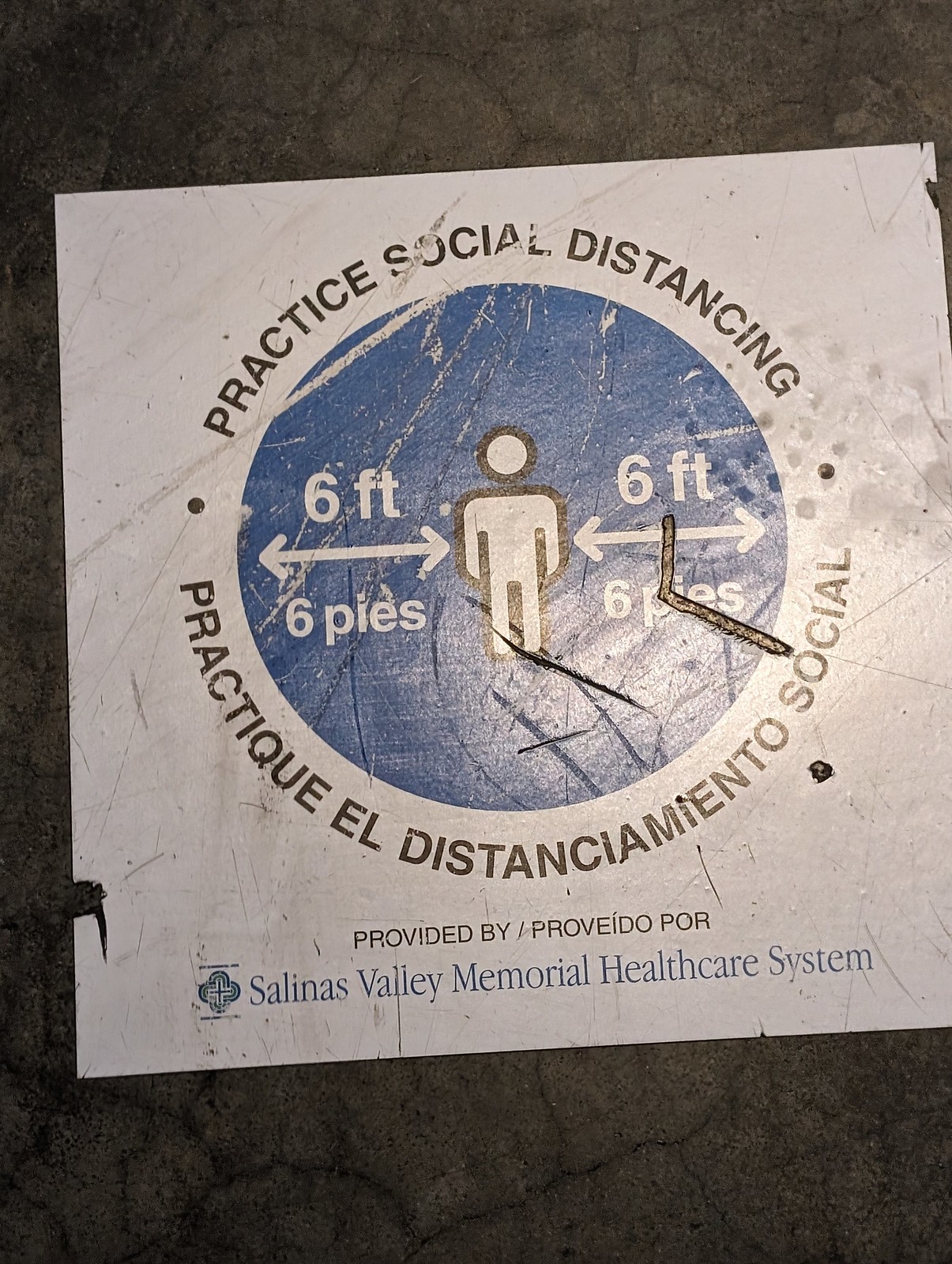The photograph features a well-worn sign adhered to a dark gray, cracked wall. The distressed white sign, torn especially on the bottom left and top right corners and heavily scuffed throughout, is still legible. Central to the sign is a blue circle containing a stick figure, bordered in black, reminiscent of the universal restroom symbol for men. The figure is flanked by arrows and text that reads "six feet" on each side, highlighting the need for social distancing. Below the arrows, the text "seis pies" is displayed on both sides of the circle. Encircling the blue area, the upper part of the white background reads "practice social distancing" in black text, with the Spanish translation "practique distanciamiento social" written similarly at the bottom. The sign also notes its provider, stating "provided by" in black and "Salinas Valley Memorial Healthcare System" in blue, accompanied by the healthcare system’s logo to the left. It appears to have endured significant foot traffic, evidenced by scratches and a noticeable footprint, suggesting it was originally placed on the floor.